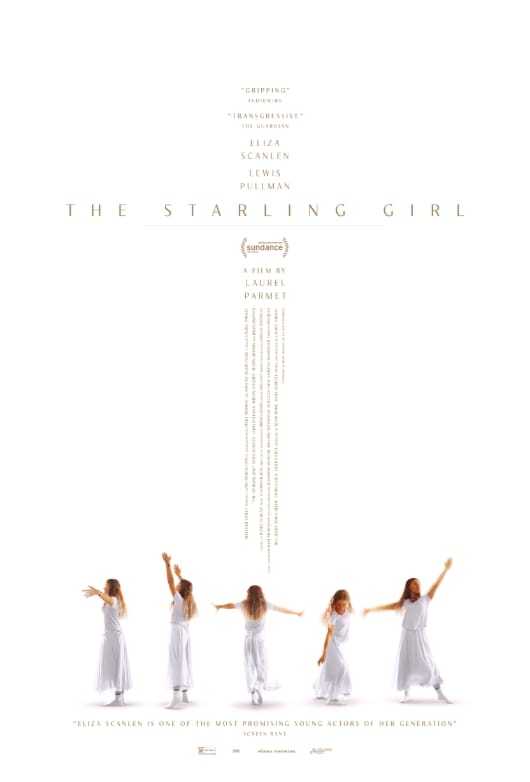This color movie poster for "The Starling Girl" prominently features a series of five photographs of the same young woman, Eliza Scanlon, performing a sequence of dance moves or movements at the bottom. She is dressed in a flowing white dress with white socks against a white background. In the first position, on the far left, she stands with her long hair cascading down, facing left with her arms stretched out in front of her. In the second image, she maintains a similar body position but has her arms raised directly upwards. The third image captures her from the back, with her arms outstretched wide on either side. Moving to the fourth position, she faces forward, bending slightly with her right arm reaching down towards the ground and her gaze following. In the final image on the far right, she stands upright, right arm extended sideways and left arm reaching to the sky, her eyes fixed on her raised hand.

Above these images, the text "The Starling Girl" is boldly featured, accompanied by the Sundance logo and the words "A Film by Laurel Parmé." Two critical quotes at the top describe the movie as "gripping" and "transgressive," and the names of the stars, Eliza Scanlon and Lewis Pullman, are prominently displayed. Additionally, a quote beneath the photographs praises Eliza Scanlon as "one of the most promising young actors of her generation," attributed to Screen Rant.